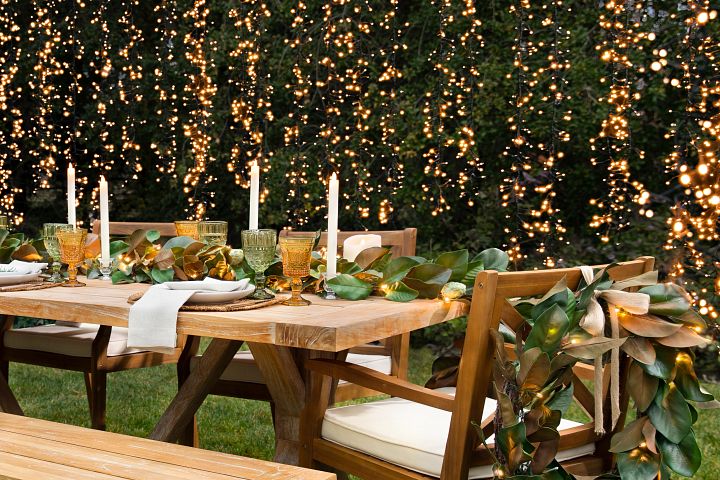This image depicts an exquisitely decorated outdoor dining area set against a backdrop of tall hedges laced with multiple strings of twinkling white lights. The focal point is a wooden table, surrounded by three visible chairs with white padding—two on the far side and one at the end closest to the viewer—and a bench on the near side. The table, evoking a cozy autumnal ambiance, is elegantly set with place settings that include plates, silverware, napkins, and two types of glasses—green and amber-colored—at each spot. The table is adorned with an array of lit candles and draped with lush greenery and decorative leaves that extend to the chairs, enhancing the festive atmosphere. The setting, possibly intended for a special occasion like a wedding or baby shower, is completed by the grassy ground beneath, adding to the overall sense of a secluded, picturesque backyard, reminiscent of a scene from a Better Homes and Garden magazine.